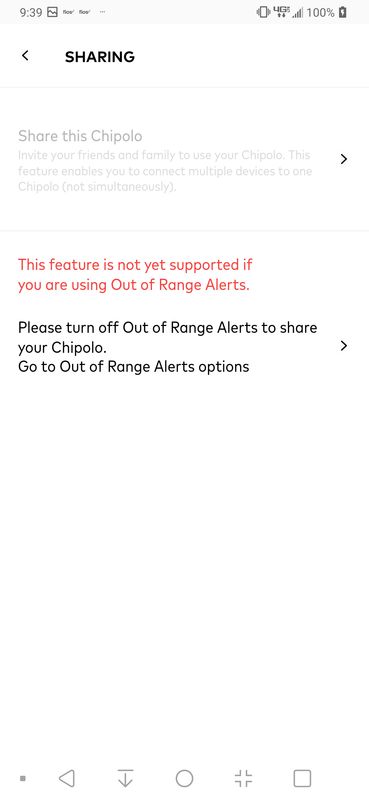The image displays a digital interface on a cell phone screen. At the top of the screen, the time is shown as "9:39" and there is a gallery icon on the left. In the top right corner, a connection icon and 100% battery life are visible. The background of the screen is predominantly white.

Below the primary navigation bar, there is a black tab with the word "Sharing." Underneath this tab, there's a small sentence in light gray text that says, "Share this Chipolo." Below the gray text, a red notification states, "This feature is not yet supported if you are using out of range alerts." Further down, there is instructional text urging the user to turn off out of range alerts to enable sharing. The instruction reads, "Please turn off out of range alerts to share your Chipolo. Go to Out of Range Alerts options," accompanied by a clickable arrow.

The lower part of the screen features icons for navigation: a dot, a sideways triangle, a downward arrow, a circle, a fullscreen option, and, in the bottom right corner, a square icon. The interface appears clean and simple, with plenty of white space ensuring readability.